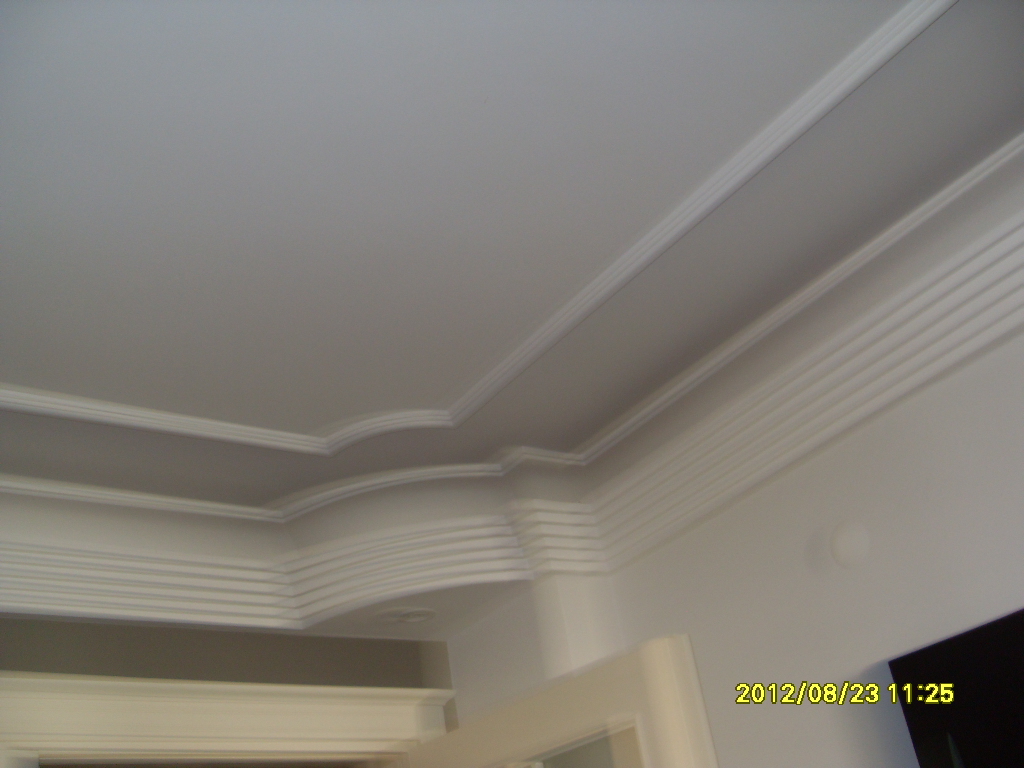This image captures the corner of a room, focusing on its ornate architectural details. The ceiling, which is off-white or light gray, features intricate crown molding with delicate striations and indentations. This molding creates a concave, circular corner rather than a standard 90-degree angle, adding elegance to the design. The top edge of the wall hosts a single white rail, similar in color to the ceiling, which continues seamlessly with the molding. Below, cream-colored kitchen cabinets with a multi-pane glass door are visible, one of which is ajar. Just beneath the open door, what appears to be part of a black TV screen is discernible in the bottom right corner. The image also contains a timestamp in yellow, indicating "2012-08-23 11:25". The photograph is slightly blurred and shows no people, animals, or plants, emphasizing the room's intricate trim work and cabinetry.